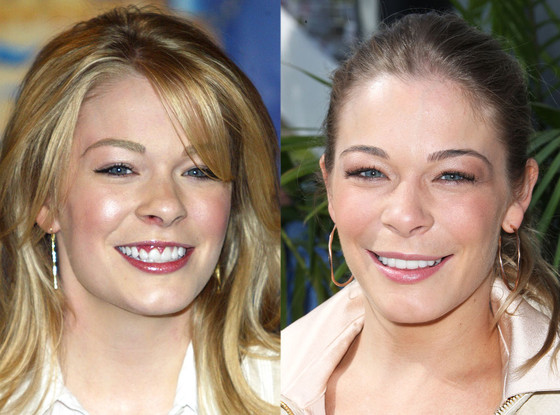This is a detailed photograph featuring a famous singer, likely LeAnn Rimes, and it presents a before-and-after comparison of her appearance. The image consists of two closely cropped headshots, showing only their faces and necks, with distinctive facial similarities suggesting they are the same person.

In the left photo, the singer has long, combed-out blonde hair with loose waves and side bangs. She is smiling broadly, revealing both her upper and lower teeth and even her top gums. Her smile is accentuated by bold red lipstick. She wears a white collared shirt and a dangling long earring visible on the right side of the image.

On the right, the singer's hair is slightly darker and tied back, giving a clearer view of her facial features. She smiles less broadly, revealing only her top teeth. Her earrings in this image are copper-colored hoops. She is dressed in a white collared top with a zipper. Both images clearly show her blue eyes and short nose.

The side-by-side comparison highlights changes in her hairstyle and dental appearance, capturing the transformation in her smile and overall look.